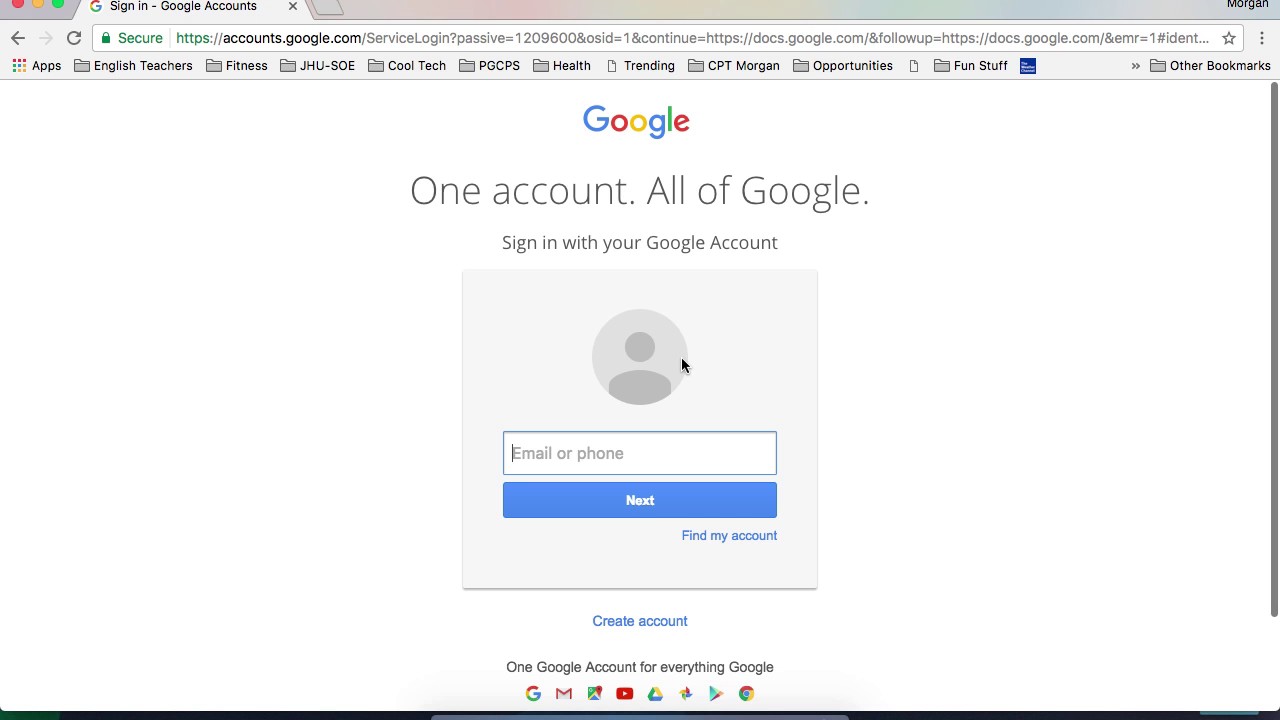The screenshot depicts an Apple electronic device displaying a web browser currently opened to the Google sign-in page. At the top left corner of the browser window, there are three familiar colored circles: the first one red, the second one yellow, and the third one green, representing the standard close, minimize, and maximize buttons. 

The browser tab is labeled with "ZenBlack Sign-in - Google Accounts," indicating that the user is on the login page for a Google account. Adjacent to the label is a green lock icon accompanied by the word "Secure," followed by "HTTPS://accounts.google.com," which illustrates that the connection to the webpage is secure and encrypted.

Dominating the center of the screen is the iconic Google logo composed of its characteristic colors: blue G, red o, yellow o, blue g, green l, and red e. Below the logo, a message in dark gray text reads, "One account. All of Google," followed by, "Sign in with your Google Account."

There is a large rectangular sign-in form beneath this text. The form starts with a gray circle icon symbolizing a user profile. Next to this icon, within a white rectangle outlined in blue, is the input field marked "Email or phone" in gray text. Beneath this input field is another rectangular button with a white background and blue text that reads "Next."

Further down are two blue link options: "Find my account" and "Create account." Finally, at the bottom of the form in black text is the phrase, "One account for everything Google."